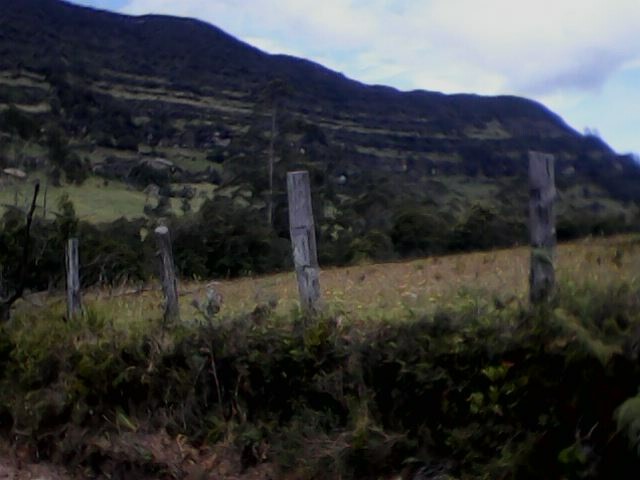The image depicts a serene, rustic landscape likely situated somewhere in Montana. The foreground is dominated by an overgrown, grassy field punctuated by four weather-worn, light gray fence posts standing vertically like aged sentinels. These posts, reminiscent of driftwood, hint at a bygone era when they might have supported wire to contain livestock. The field itself appears brownish and untamed, suggesting a space that has long been left to nature's devices.

As the eye moves past the fence, the terrain slopes gently upward into a hillside adorned with a mix of grass, brush, and trees, their colors muted by the seasonal touch of autumn. The mountain range beyond stretches into the distance, its ancient sediment lines and layered strata visible, narrating eons of geological history.

Above, the sky is a canvas of blue and white, filled with a scattering of clouds that add depth and contrast to the scene. Despite the overall darkness of the lower portion of the photo, the image still evokes an atmosphere of timeless beauty, inviting viewers to ponder the quiet stories held within this pastoral vista.